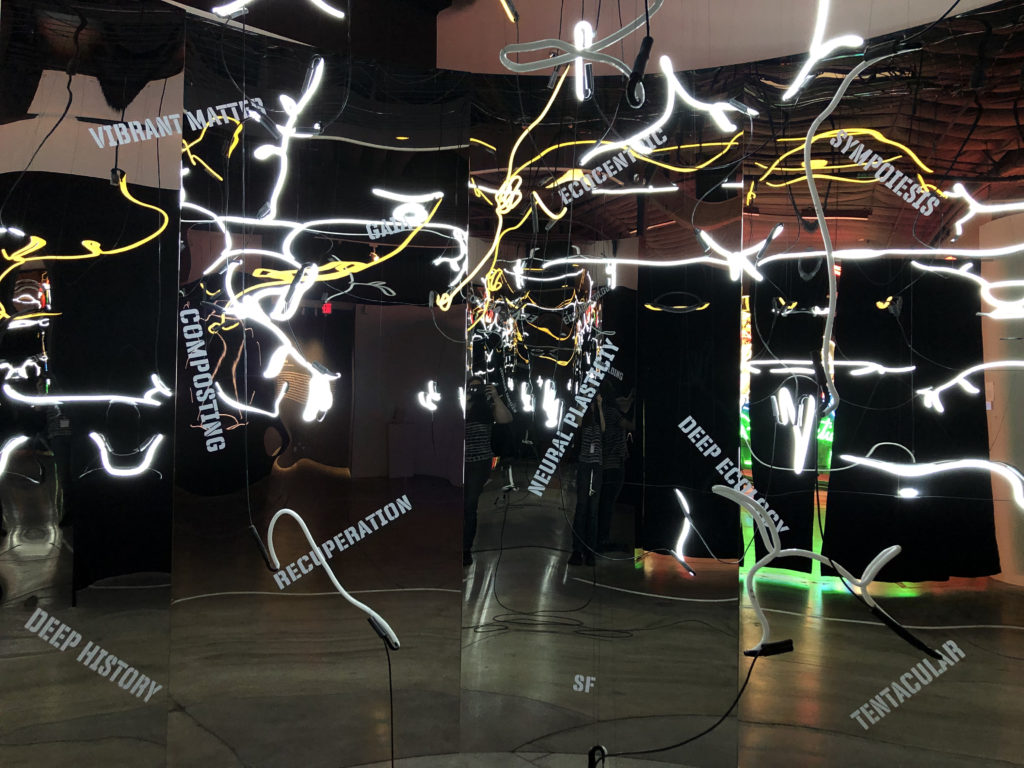This image captures an intricate art installation set inside a room with a polished, shiny concrete floor. The installation features several reflective mirrors and numerous neon white lines that depict an electrified effect. Scattered throughout the image are yellow, white, and black wires intertwined with the neon lines, adding to the complexity of the scene. Prominent words are displayed across the mirrors and other parts of the installation, including "Deep History" in the bottom left corner, "Vibrant Matter" at the top left, "Composting" in the middle left, "Recuperation" beneath that, "Neuroplasticity" in the middle, "Sympoiesis" at the upper right, and "Tentacular" in the bottom right. An intriguing element is the reflection of a woman holding a camera, capturing this dynamic installation, which emphasizes themes of deep ecology, vibrant matter, and eco-centrism.